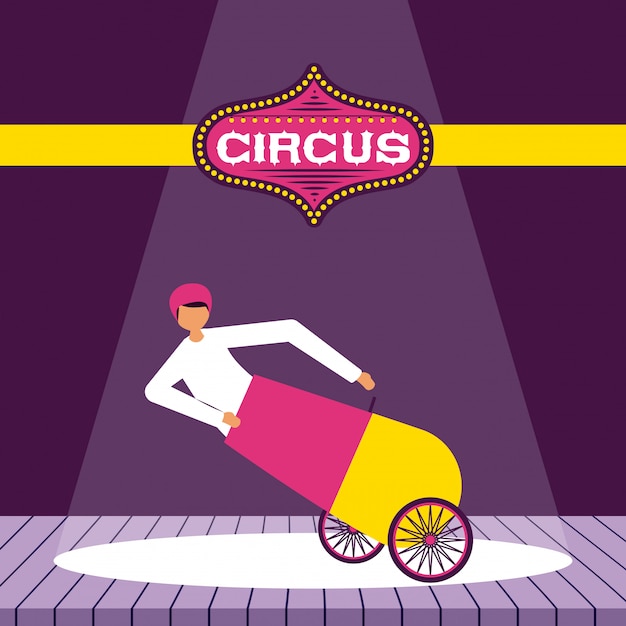The image is a simple yet vibrant graphic design illustration, predominantly featuring shades of pink, purple, yellow, and white. It depicts a performer with slightly tan brown skin and a long-sleeved white shirt, wearing a plain pink cap, about to climb into an old-fashioned cannon. The cannon itself is divided into two colored segments: the front half is pink, and the rear half is yellow, with black wheels that have pink rims. This scene takes place on a lavender-colored wooden platform, indicated by lines resembling wooden planks, with a spotlight focusing on the performer and the cannon. 

The background is a deep purple, providing a dramatic contrast to the brightly colored elements in the foreground. At the top center of the image is a stylized circus logo. The logo is inscribed in white, Las Vegas-style text within an elongated teardrop shape that resembles an onion. This shape is pink, bordered in black, and adorned with yellow dots resembling lights. A yellow stripe extends horizontally from each side of the logo towards the image's edges, emphasizing the vivid and playful circus theme. 

The illustration, carrying a flat 3D cartoonish style, conveys dynamic action and anticipation, clearly setting the stage for a thrilling circus performance.